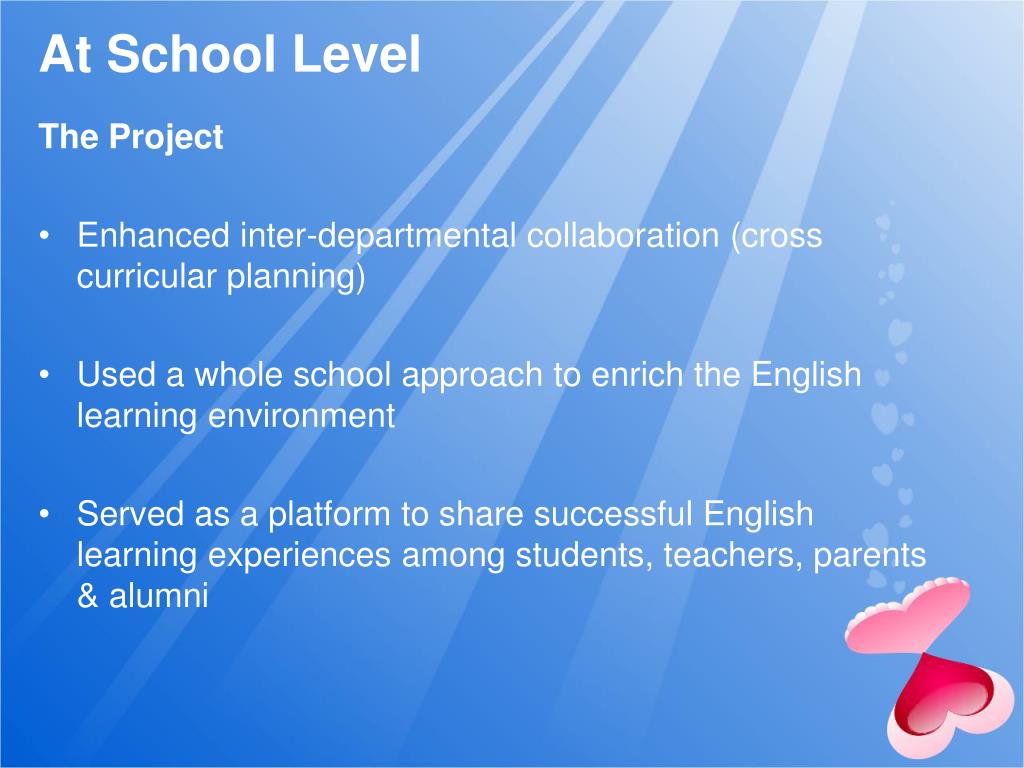The slide features a light blue background with lighter blue rays streaming down from the top. A red, pink, and white heart graphic adorns the lower right-hand corner. The text, in white font, begins with the heading "At School Level" at the top left, followed by the subheading "The Project." Below, three bullet points outline key aspects of the initiative: "Enhanced Interdepartmental Collaboration (Cross-Curricular Planning)," "Used a Whole School Approach to Enrich the English Learning Environment," and "Served as a Platform to Share Successful English Learning Experiences Among Students, Teachers, Parents, and Alumni." The slide effectively conveys a comprehensive strategy to improve English learning through collaboration and community engagement.